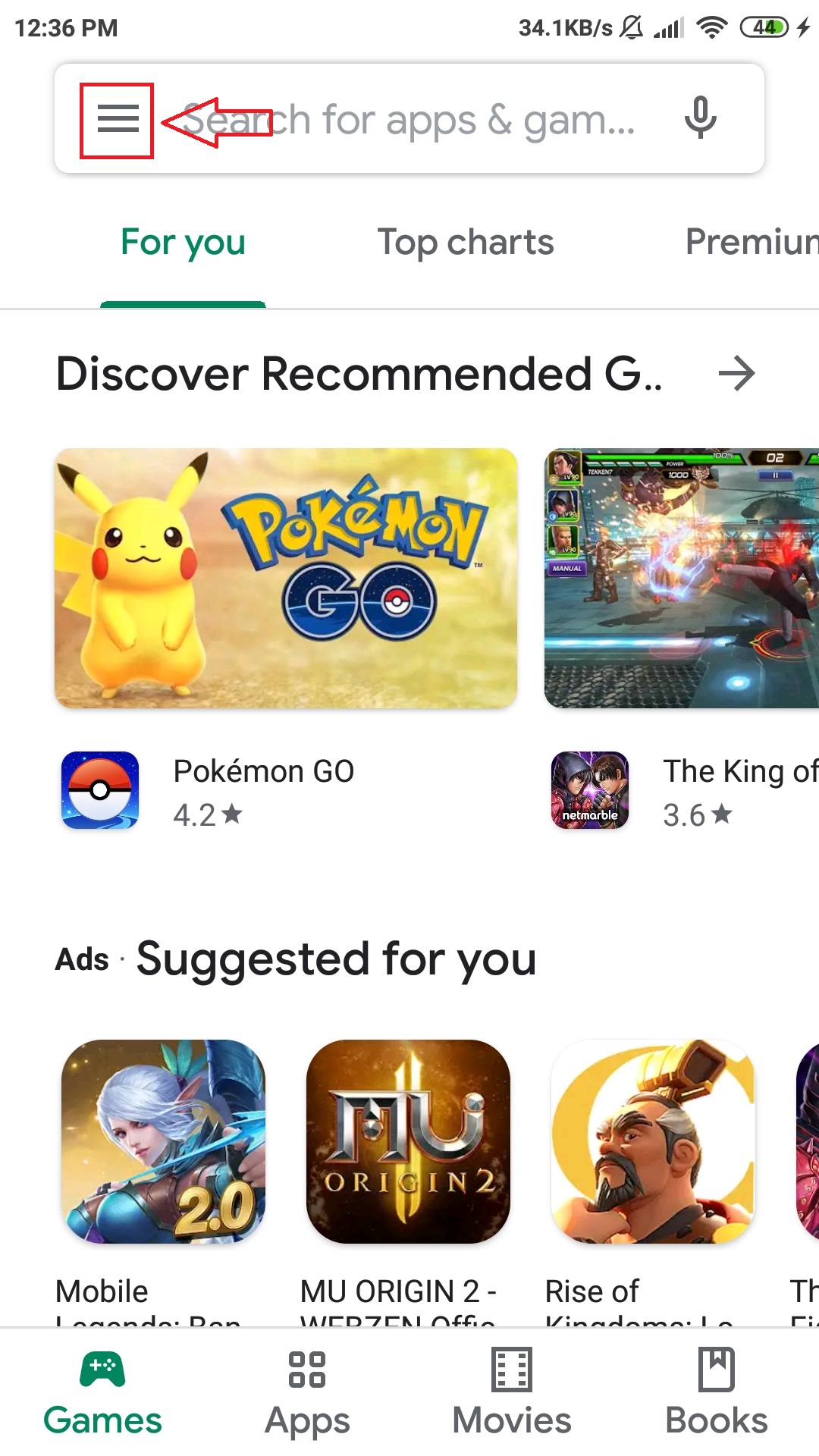### Cleaned and Detailed Caption:

This image depicts a screenshot from a smartphone. On the top left, the time is displayed as 12:36 PM, while on the right, the data usage is shown as 34.1 KB. The notification bell icon is crossed out diagonally, indicating that notifications are silenced. The status bar also shows cellular signal bars, a Wi-Fi icon, and a battery icon at 44% capacity, which is currently charging.

The image has been edited with red markings. Across the search bar, located near the top, there's a red outline and an outlined red arrow pointing towards the search bar, which contains three horizontal lines within it. Below the search bar, the navigation menu includes options such as "For you," "Top charts," and "Premium." The currently selected option is "For you," highlighted in green with a green underline, while the other options are in black.

Underneath this navigation menu, there's text that reads "Discover recommended," with an icon depicting the letter "G" followed by three dots, and a right arrow symbol. Below this, a list of app recommendations is partially visible, including titles such as "Pokémon Go" rated 4.2 stars, partially cut-off titles like "The King of..." rated 3.6 stars, and other suggestions. The word "Add" and "Suggested for you" are also visible.

At the bottom of the screen, there's a horizontal menu featuring icons and labels for various categories: "Games" (highlighted in green with a gaming icon), "Apps" (four squares forming a larger square), "Movies" (represented by a film icon), and "Books." The "Games" category is currently selected.